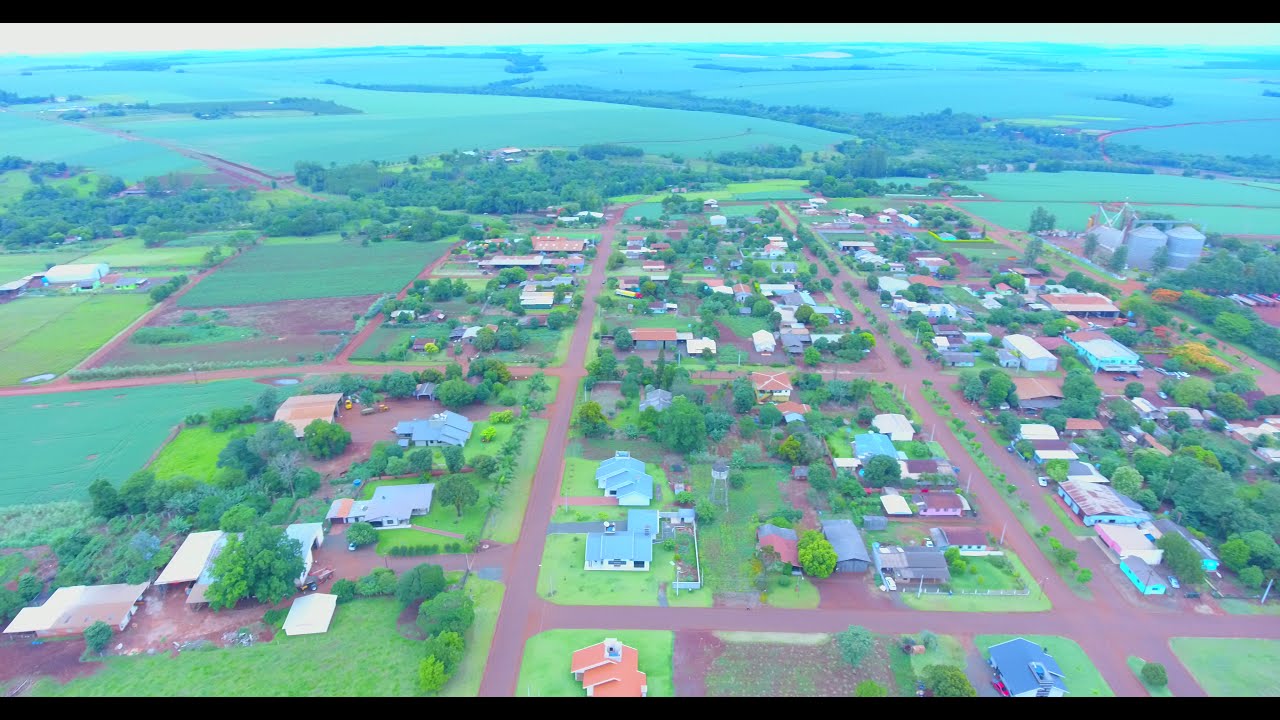The drone shot captures a quaint, very wet, rural village characterized by a diverse array of houses with eclectic roofs of blue, red, brown, and white. These homes are seemingly built as needed, contributing to varied architectural styles. The village, nestled within expansive green plains, features a large water tower on the right-hand side, amidst an abundance of trees and grass. The center of the image reveals a cluster of ranch-style buildings, intersected by dirt roads forming a crisscross pattern. Farmland dominates the left side and top of the image, punctuated by patches of dirt and vibrant greenery. The scene, devoid of oceans and framed by a unique black border at the top and bottom, offers a picturesque view of this rural community surrounded by open fields, resembling a serene Midwest landscape from above.